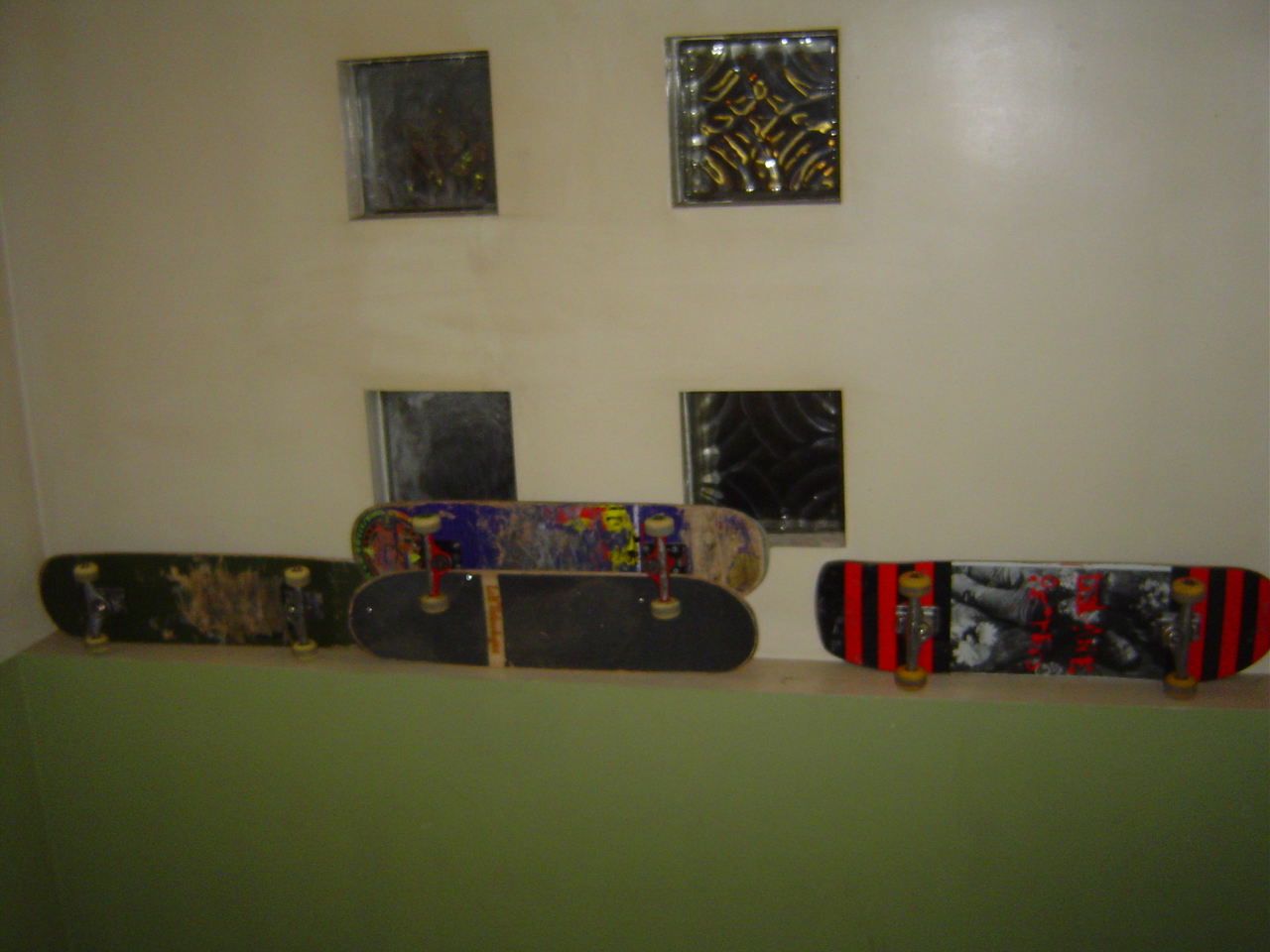In the image, four skateboards rest against a white wall, which appears dirty in spots, adding a touch of grit to the scene. These skateboards are placed on a light, dull green shelf. The arrangement is interesting: three of the skateboards have their bottom sides facing the camera, showcasing scraped-off artwork, while the fourth, positioned at the bottom of the middle stack, has its top side visible. Above the skateboards, there are four small, square windows featuring decorative, thick glass blocks. These blocks, typical of basement settings, obscure visibility both in and out, hinting at a slightly industrial environment. The overall scene exudes a sense of urban decay and casual disarray.